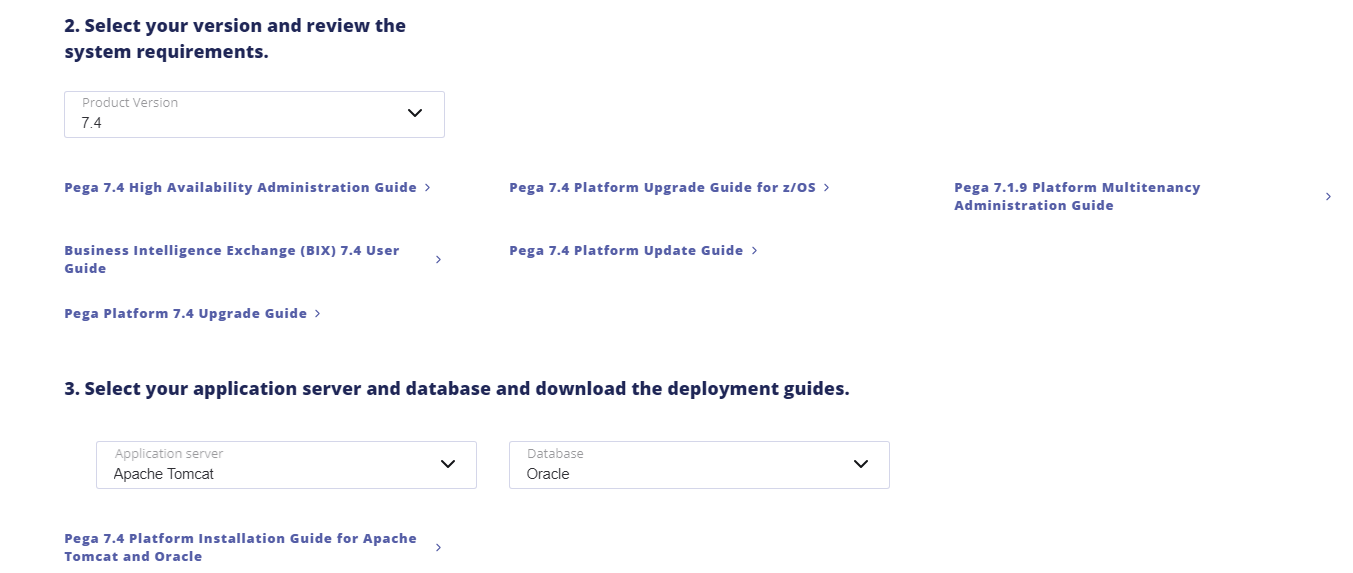This screenshot captures a partial view of a web page designed for server setup, missing the company or product name due to the absence of the header and footer. In the upper left-hand corner, the number "2" indicates a step in a sequence, suggesting this is only a part of a multi-step process. Step 2 instructs users to select their version and review the system requirements. This is followed by a dropdown menu for making the selection, and a description listing various guides: "APEGA 7.4 High Availability Administration Guide" and "Business Intelligence Exchange (BIX) 7.4 User Guide."

Below, step 3 guides users to select their application server and database, and to download the deployment guides. Apache Tomcat has been pre-selected for the application server, while Oracle is chosen for the database in corresponding dropdown boxes.